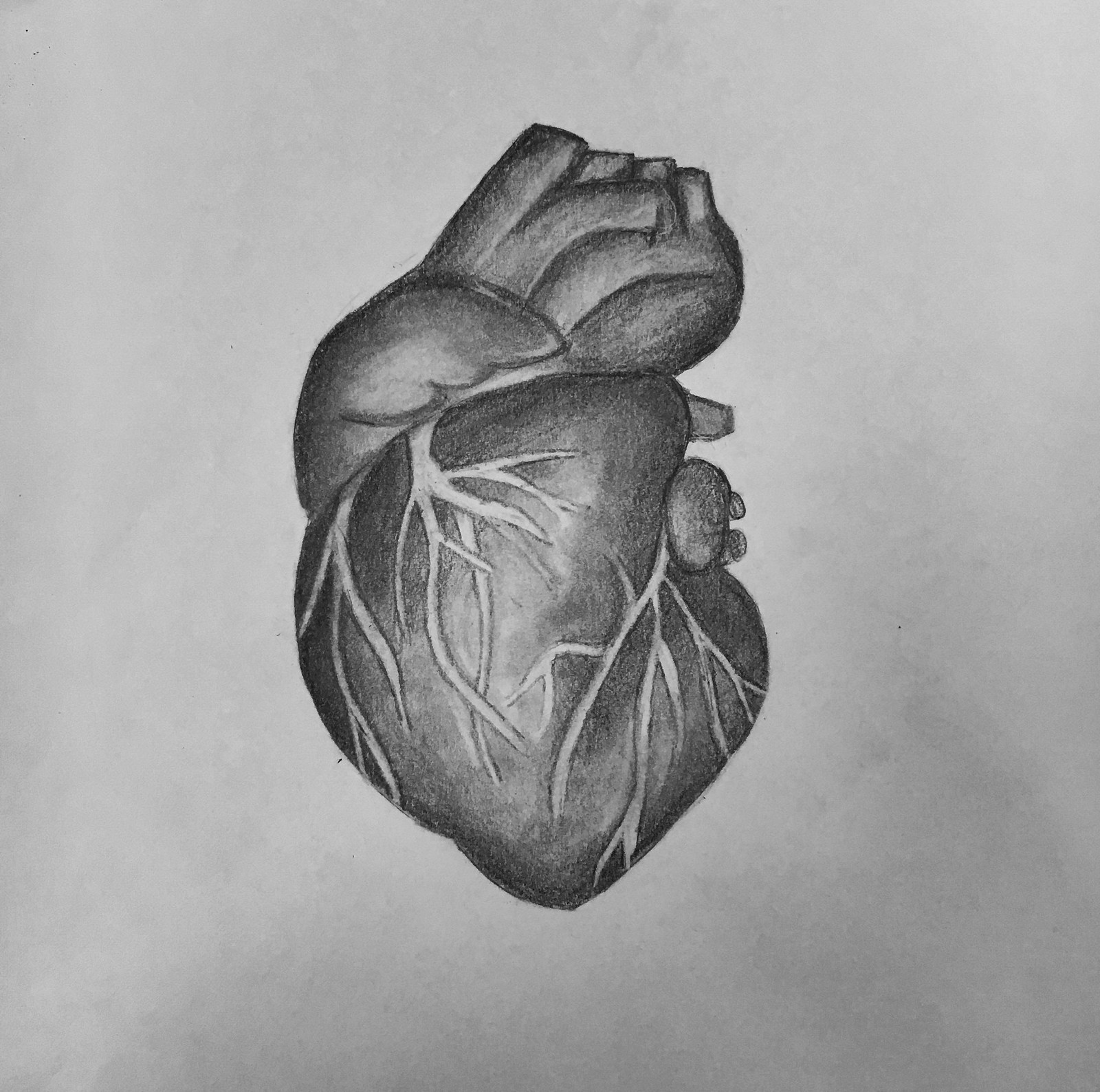A highly detailed and realistic drawing of a human heart is central to the image, positioned on a pristine white piece of paper. The drawing, created with either varying shades of gray and black colored pencils or a regular pencil, meticulously captures the complexity of the heart with visible valves and aortas intricately connected. The heart's primary sections are adorned with finely drawn veins and arteries, presented through delicate gray shading that blends seamlessly with the white of the paper. These veins and arteries depict a naturalistic flow, enhancing the lifelike quality of the image. As the drawing extends to the various connecting points that feed into the body's circulatory system, the shading intensifies, creating a striking contrast and emphasizing the depth and realism of the heart's anatomical structure. The zoomed-in perspective focuses solely on the drawing, omitting any surrounding context, and highlighting the artist's precision and attention to detail.